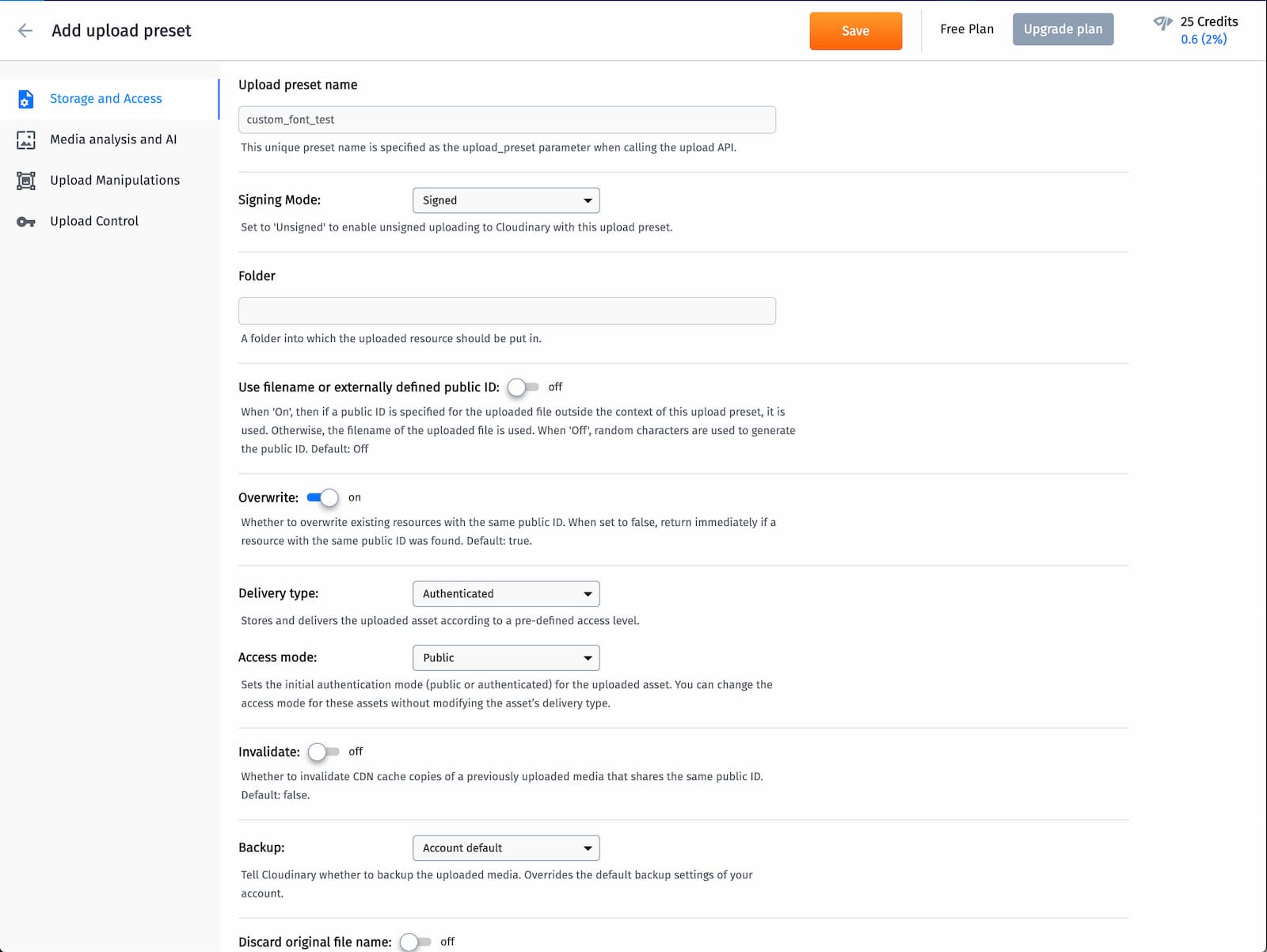The webpage features an interface focused on configuring upload presets. At the top of the page, there are options to "Add Upload Preset" and a gray left arrow icon for navigation. Below this, a blue section labeled "Storage and Access" with an accompanying icon is displayed. Other options like "Media Analysis and AI," "Upload Manipulations," and "Upload Control" are written in gray beneath it.

An orange rectangular "Save" button is prominently featured at the top right corner, accompanied by "Free Plan" in gray text and a gray rectangular "Upgrade Plan" button. The page also includes an indicator showing "25 Credits" and a quantitative status of "0.6 (2%)" in blue.

Centrally, there's a section for "Upload Preset Name," with a rectangular input box below it labeled "Custom Font Test." This section explains that this unique preset name is used as the upload preset parameter when initiating the upload API. Further down, under "Signing Mode," there is a field marked "Sign" with a down-arrow icon in black, indicating a dropdown menu.